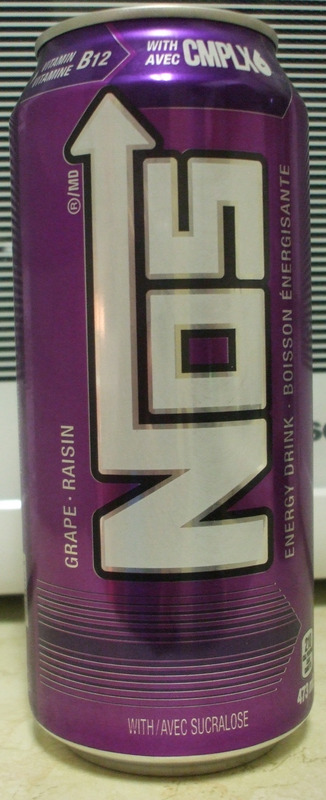This image showcases a close-up view of a tall, purple can. Prominently displayed on the left side of the can is the word "grape" followed by "raison," which is French for grape. At the bottom of the can, the text "with sucre," meaning "with sugar" in French, is visible. The brand name appears to be "Sun," spelled out as "S-O-N," though the letters could alternatively be read as "N-O-S" or "N-O-5." The letter 'N' features a long arrow as part of its design. Near the top of the can, "avec C-M-P-L-X-6" and "B-12," referring to the inclusion of vitamin B-12, are inscribed. The can is placed on a light-colored surface, with what seems to be a window with numerous blinds in the background. The view beyond the blinds is dark, adding contrast to the scene.